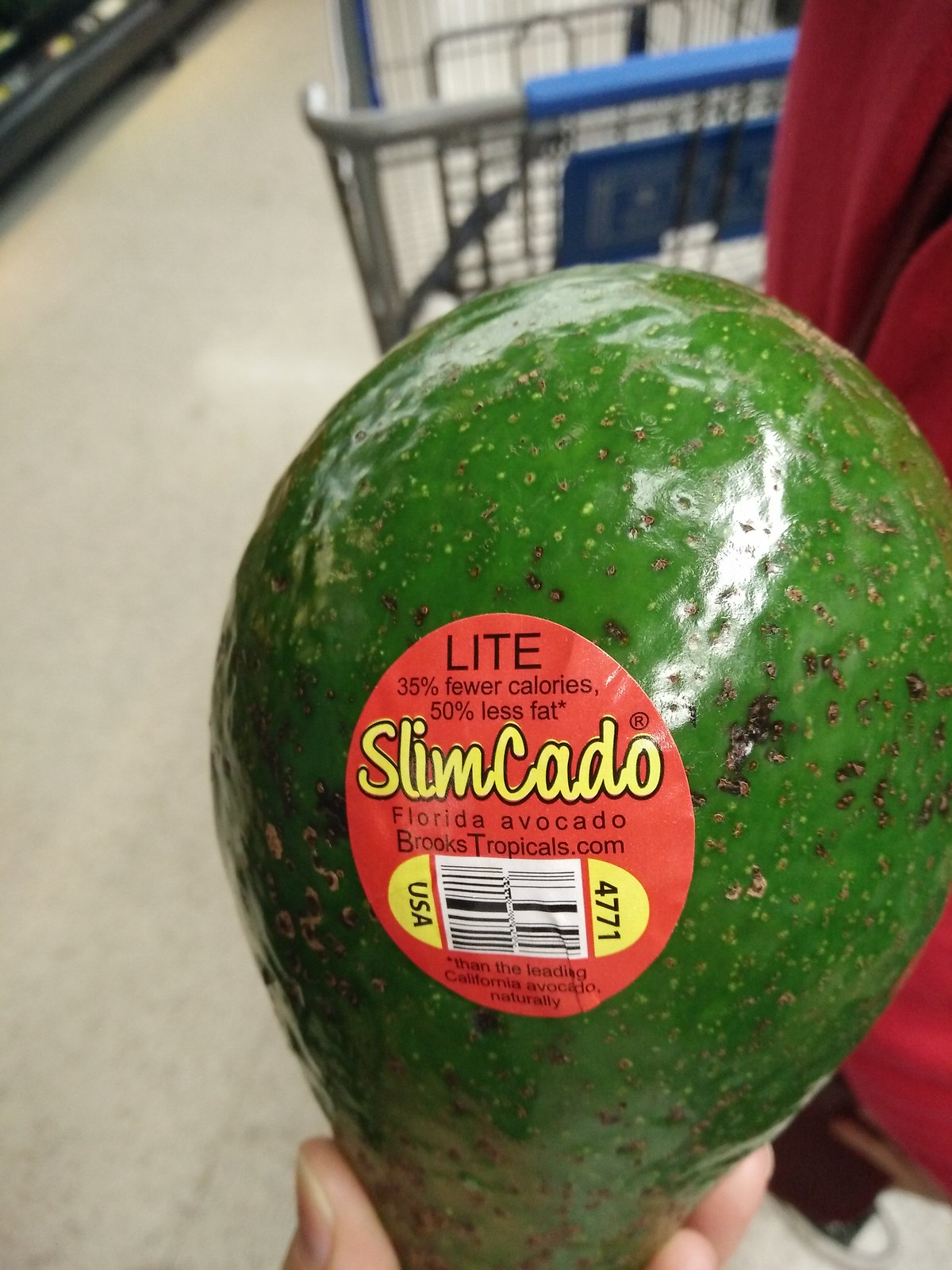The image depicts a close-up of a bright green, shiny Florida avocado being held between the thumb and fingertips of someone's hand. The avocado is prominently featured in the foreground, showing a smooth surface with small brown dots and an overall lighter green hue. A red label is affixed to the avocado, bearing detailed information which includes: "Light, 35% fewer calories, 50% less fat, Slim Kato, Florida Avocado, brookstropicals.com, USA, 4771." The label also states, "*Leading California avocado naturally." In the background, a grocery store aisle is visible, with white flooring and a slightly blurred person dressed in red pushing a blue and silver shopping cart.